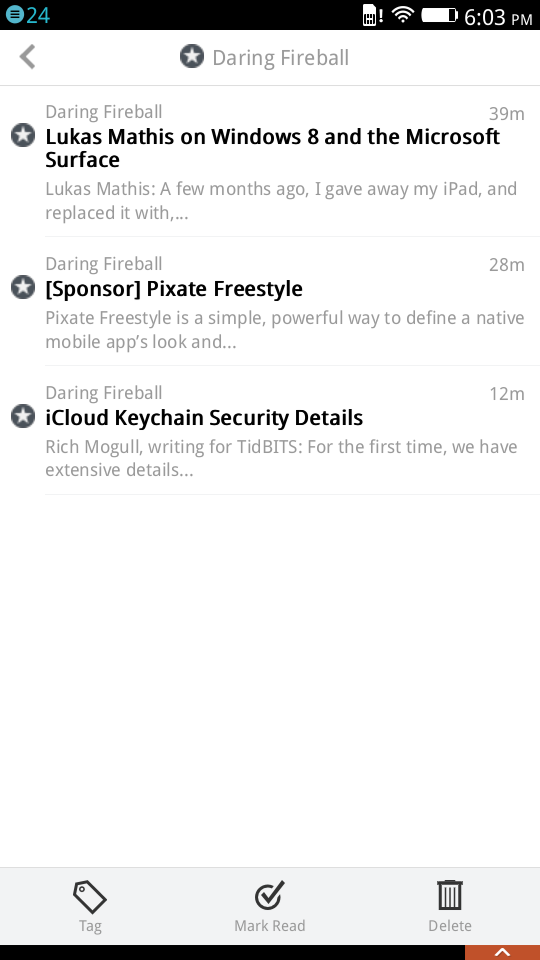A smartphone screenshot displays a content list from a mobile application. The screen features a black header with the number "24" in aqua, a WiFi reception signal, and a battery icon indicating approximately 85% charge. The current time is displayed as 6:03 PM.

At the top left of the screen, there is a back button, followed by a star icon and a black circle. The title "Daring Fireball" is prominently displayed. Below this header, a list of three entries is presented, each marked by a star and a black circle.

1. **Daring Fireball: Lucas Mathis on Windows 8 in the Microsoft Surface**
   - **Author:** Lucas Mathis
   - **Description:** "A few months ago, I gave away my iPad and replaced it with..."
   - **Duration:** 39 minutes

2. **Daring Fireball: Sponsor (Pix8 Freestyle)**
   - **Description:** "Pix8 Freestyle is a simple, powerful way to define a native mobile app's look and..."
   - **Duration:** 28 minutes

3. **Daring Fireball: iCloud Keychain Security Details**
   - **Author:** Rich Mobile, writing for Tidbits
   - **Description:** "For the first time, we have extensive details..."
   - **Duration:** 12 minutes